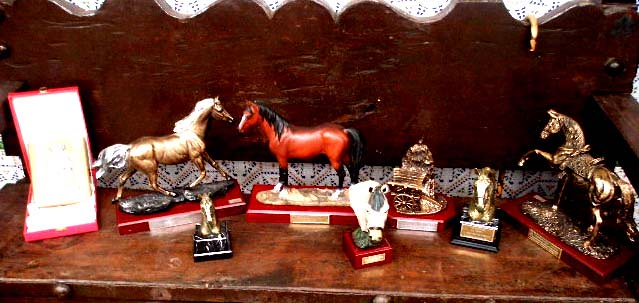In this detailed photograph, we see an old, dark-stained wooden table adorned with a variety of horse-themed knick-knacks. The scene is set against a wooden backdrop, hung on a wallpapered wall. There are seven objects in total, including four full-bodied horse figurines and two horse head busts, along with what seems to be a model of a cabin. On the far left, there is an open red jewel box containing a square golden object, though the details are obscured due to blown-out highlights.

Starting from the left, we see a golden horse with a silver mane and tail depicted prancing across black rocks. In front of it is a golden horse bust on a small black square pedestal. Next to this is a red chestnut horse with a white marking on its face, standing in a neutral position with a black mane and tail. Before this statue, there is a white horse bust with a gray mane mounted on a red wooden block, featuring a golden plaque. Adjacent to it stands an indeterminate golden object on a similar red stand with a golden plaque, possibly a cart as a wheel is visible. Further to the right is another golden horse bust on a square black block with a golden plaque. Finally, at the far end, there is a bronze horse statue with its leg raised and ears pointed forward, mounted on a reddish wooden block with a golden plaque. The arrangement evokes the look of an old hutch or dresser, creating a nostalgic tableau of equestrian artistry.